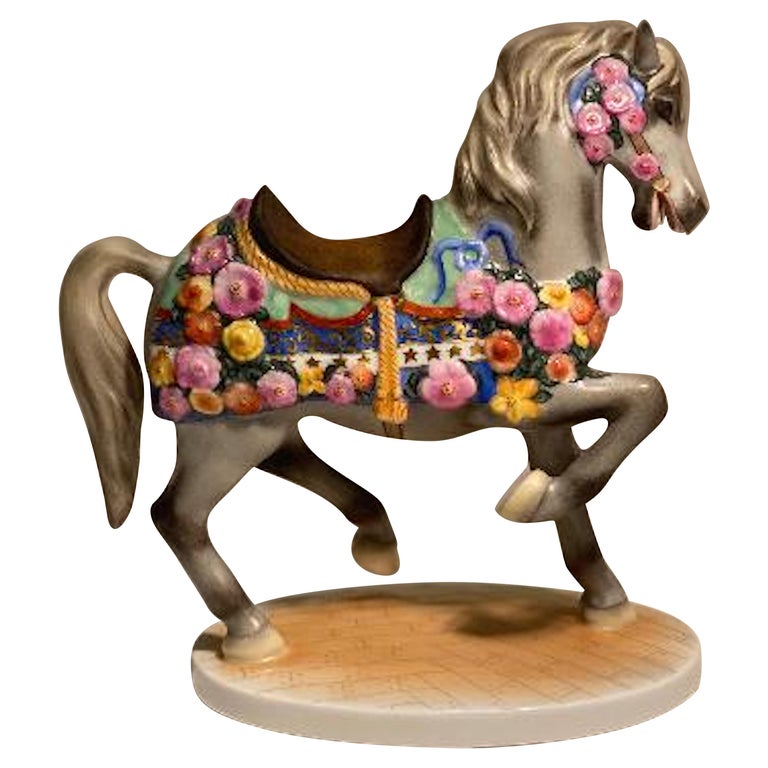The image features a small decorative statue, likely made of porcelain or plastic, depicting a prancing gray horse with an ivory-colored hoof on each foot. The horse's front right and rear left legs are lifted, accentuating its dynamic pose. It sports a glistening golden mane and tail that hangs slightly to the left. The horse is adorned with a richly detailed bridle and saddle, complete with a turquoise blanket edged in red trim and another larger dark blue blanket below, featuring white horizontal lines and gold five-point stars. The ensemble includes intricate flower decorations, showcasing pink, yellow, blue, and peach-colored blooms, possibly camellias, situated near the horse’s ear and around its chest. Additionally, the saddle is embellished with a decorative gold rope and a tassel hanging down from its center. The statue is affixed to a small, circular base with a beige top crisscrossed by brick-like lines and a light gray rim. The horse's open mouth and poised stance suggest a spirited trot, making it an ideal decorative piece, perhaps intended for a young girl.